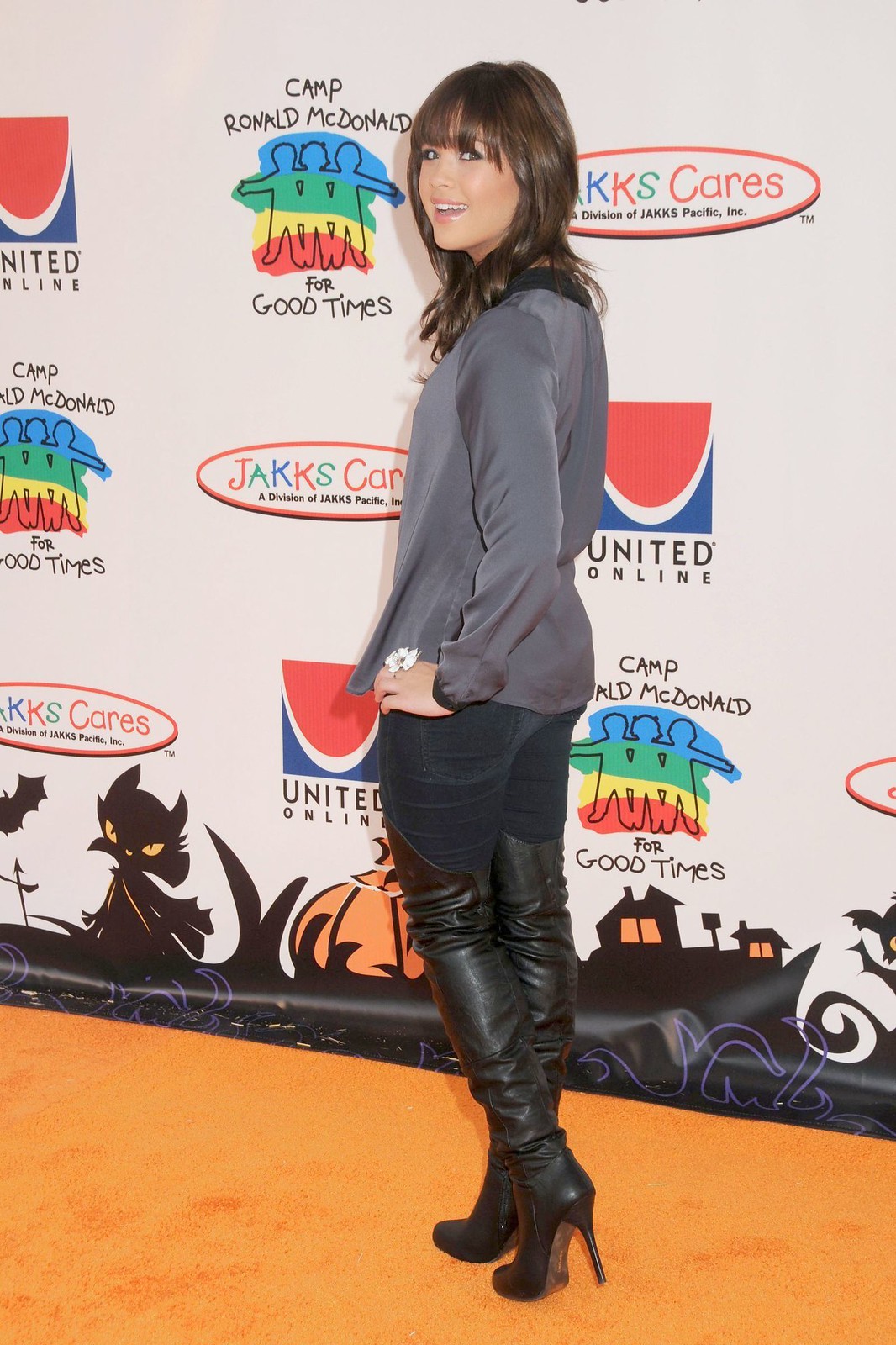In this image, we see a young Caucasian woman, likely an actress or celebrity, posing on an orange carpet at a charitable event. She has shoulder-length brown hair with bangs, and she is smiling back at the camera, revealing her top row of teeth. Her stance is slightly turned away, offering a side and back view with her left hand resting on her hip, showcasing a ring with a white flower on it. 

She is dressed in knee-high, black leather high-heeled boots, paired with dark blue jeans, and a long-sleeved, silky gray jacket. The backdrop of the event features a large white banner adorned with multiple logos and advertisements, including "Camp Ronald McDonald for Good Times," "JAKKS Cares" (a division of JAKKS Pacific Inc.), and "United Online." The banner is festively decorated at the bottom with Halloween-themed images including a black cat, a bat, haunted houses, and Jack-O-Lanterns, emphasizing the seasonal theme of the event.